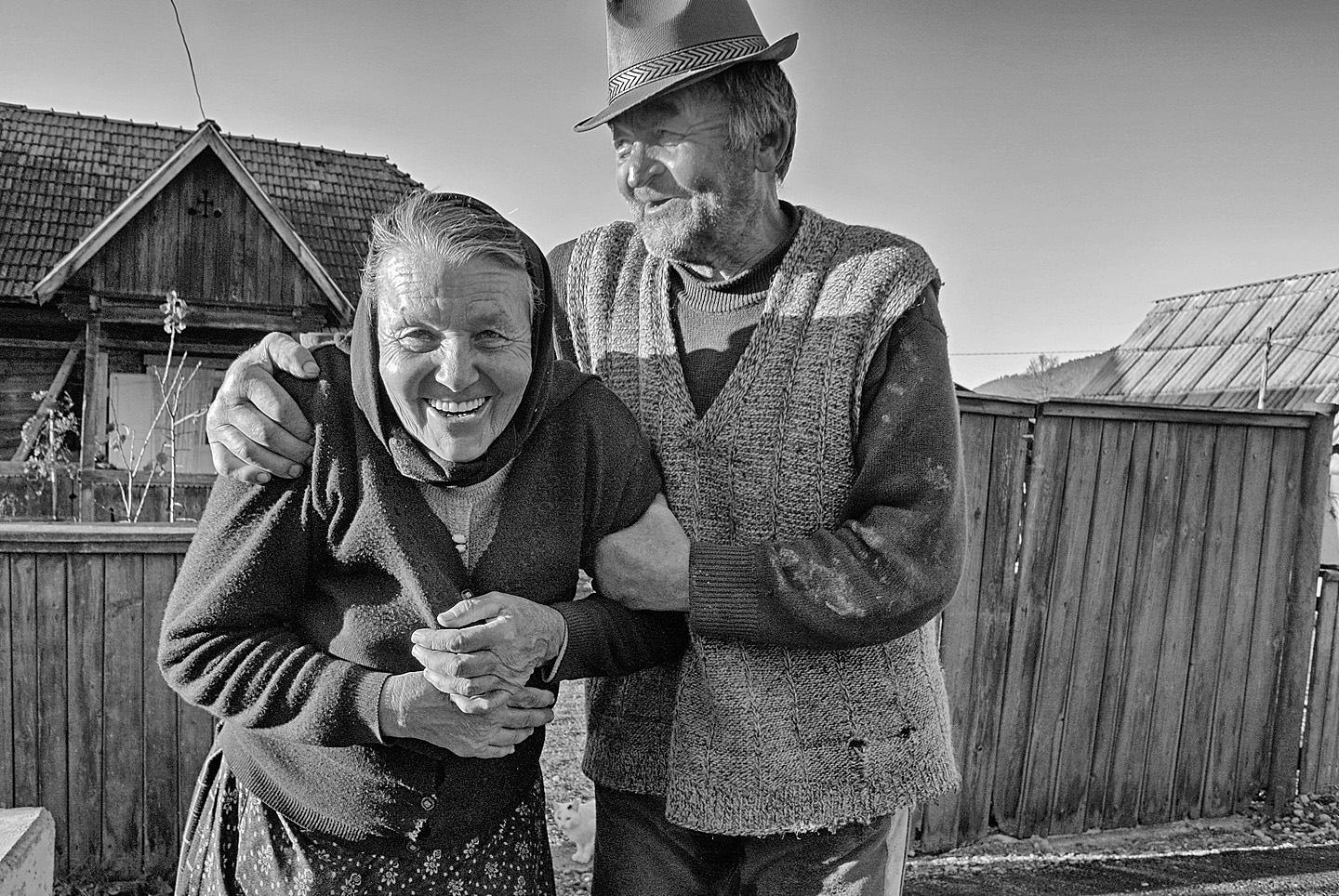This black and white vintage photograph, likely from the late 1930s or 1940s, captures an elderly man and a woman standing closely together in front of a wooden house and fence. The man, who has gray hair and a slightly unshaven face, is wearing a fedora hat with a band, a sleeveless vest over a long-sleeved sweater, and dark pants. His left arm is wrapped around the woman's upper arm, and his right hand rests on her shoulder. The woman's grayish hair is neatly combed to the right, partially covered by a kerchief or hood, and she is smiling warmly at the camera, wrinkles around her eyes visible. She is dressed in a dark cardigan sweater and a floral printed skirt. Both their clothing and the setting suggest a modest, possibly Depression-era rural backdrop. The image shows a detailed view of the rustic environment, with a wooden fence varying in height and a small cottage discernible in the background to the left.